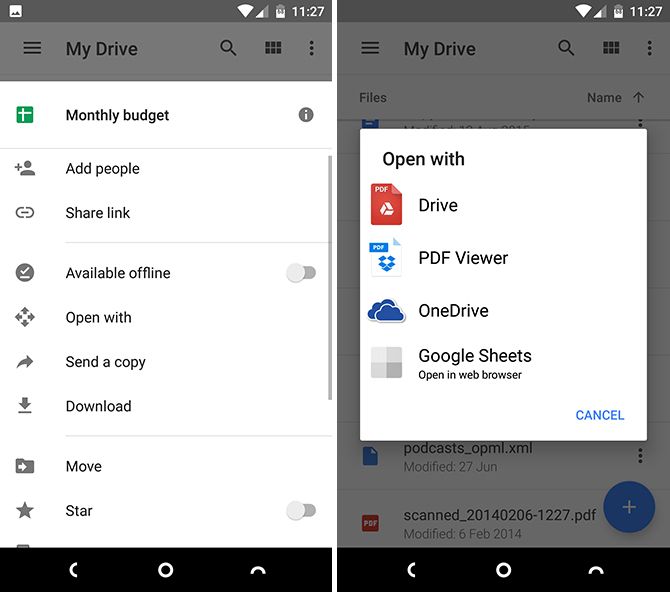In the image, there are two screenshots taken from the same Android phone, displayed side by side. The left screenshot shows a white window that has slid up from the bottom of the screen, presenting a list of action buttons. The options available in this list are as follows: "Monthly Budgets" at the top, followed by "Add People," "Share Link," "Available," "Offline," "Open With," "Send a Copy," "Download," "Move," and "Star." 

The right screenshot displays a squared window positioned in the center of the screen, with the top left corner labeled "Open With." This window provides the user with four options for opening a file: "Drive," "PDF Viewer," "OneDrive," and "Google Sheets." In the bottom right corner of the squared window is a "Cancel" button. Both screenshots have a dimmed background, revealing a list of various file names that are hard to discern due to the darkened overlay, indicating the presence of files in the background.